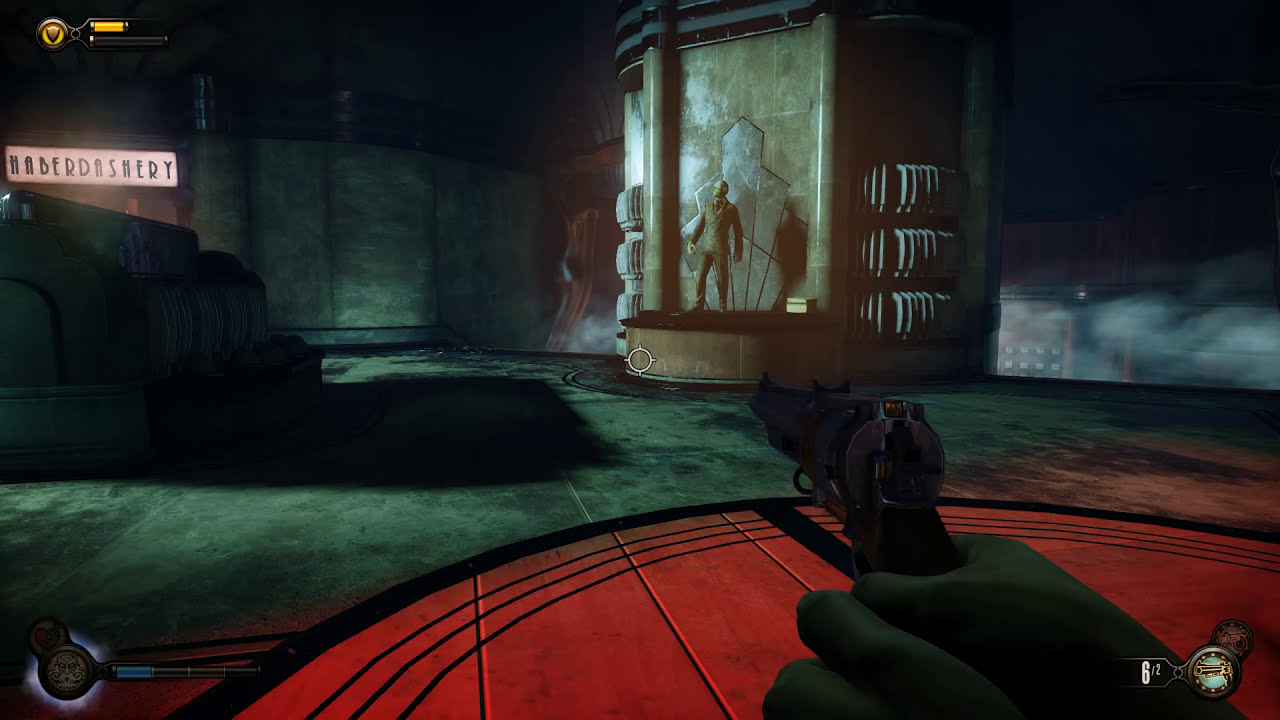In this image, which is a screenshot from a dark, synthetic video game environment, the player's perspective is in first-person view. The scene features a red circular platform on the bottom portion of the screen, comprised of wooden beams and outlined in black. A hand holding a revolver pistol is visible on the lower right, supported by the character's left hand, with the gun aimed towards a door on the back-left side of the space. A crosshair cursor, defined by a circle with four directional lines, is centered on the screen, enhancing the aim. The lower right corner includes a navigation or informational display showing a revolver icon in a grey circle with a blue background, and numbers "6/2." Additional interface elements include a grey circle with a white central portion in the bottom left, a grey circle with a red heart, and multiple health bars. The top left corner of the screen features a gold shield icon with a grey circle, accompanied by corresponding bars. The setting appears to be a shaded concrete room with intricate details. A statue of a man stands on a pedestal to the player's front right, near an entrance to another room below. Overhead, a neon sign in black font reads "HABERDASHERY," contributing to the synthetic atmosphere of the game.